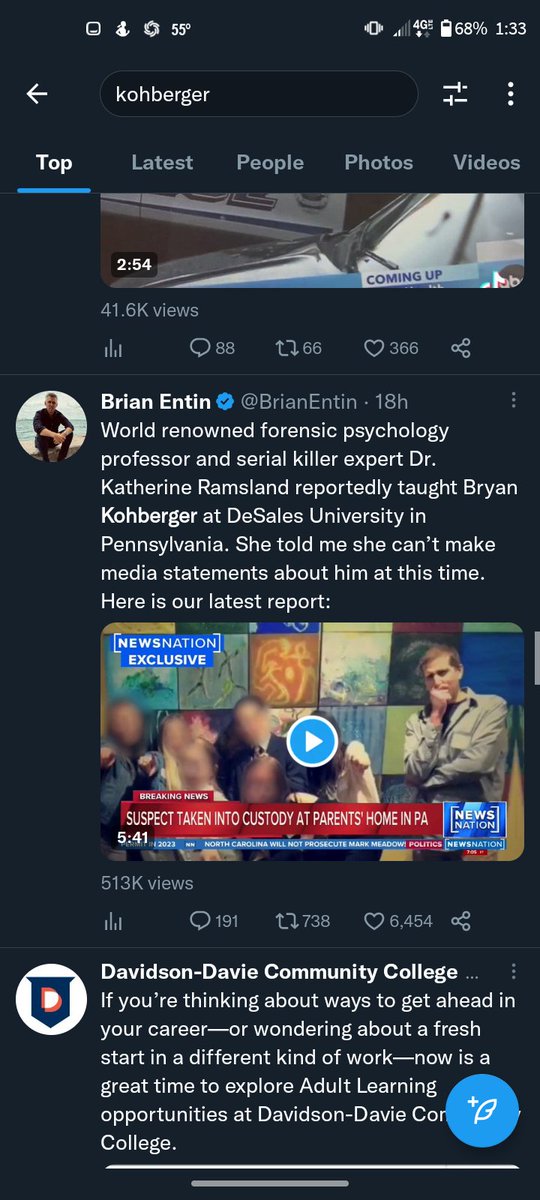In this detailed image caption, we observe a screenshot of a cell phone displaying an interface of a social app, likely Instagram. Starting at the top of the screen, the status bar reveals several icons: on the far left, there are three generic icons, while on the right, it shows the time "1:33," the temperature "55°F," and four additional icons. These include a watch icon, a 4G network signal indicator, and a battery icon indicating 68% battery life.

Beneath the status bar lies a search bar with the text "Cobra K-O-H-B-E-R-G-E-R." To the immediate right of this bar, two slider icon overlays are stacked vertically, followed by a more options icon consisting of three vertical dots.

Below the search bar is a horizontal menu bar with tabs labeled "Top," "Latest," "People," "Photos," and "Videos." The "Top" tab is underlined in blue, indicating it is the currently active tab.

The main part of the screenshot shows various content feeds from users such as Brian, Tin, and David from Davey Community College, along with indications of viewership, shares, activity, and conversations. These posts are likely sorted under the "Top" feed category, providing the most relevant or popular posts at the time.